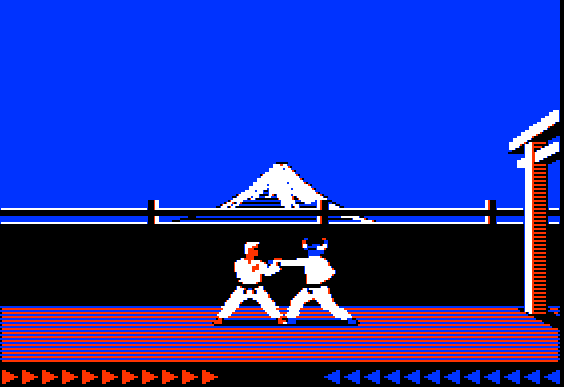In this vibrant arcade-style fighting game scene, the characters are engaged in a dynamic battle on a distinctive orange and blue striped floor. The character on the left is an orange figure donning a white robe cinched with a black belt, while the opponent on the right is a blue figure similarly attired in a white robe and black belt. The background includes a black fence directly behind the fighters, adding a layer of depth and confinement to the scene. To the right, an orange pillar supports part of a structure, juxtaposed against a white mound visible in the distance. The sky above is a clear expanse of blue, providing a vivid backdrop to the unfolding action. At the bottom of the image, a black bar features prominently with an orange line above it. Inside this bar, 11 orange arrows point to the right and 12 blue arrows point to the left, possibly indicating directional controls or gameplay mechanics. This setting encapsulates the intensity and visual appeal typical of retro fighting games.